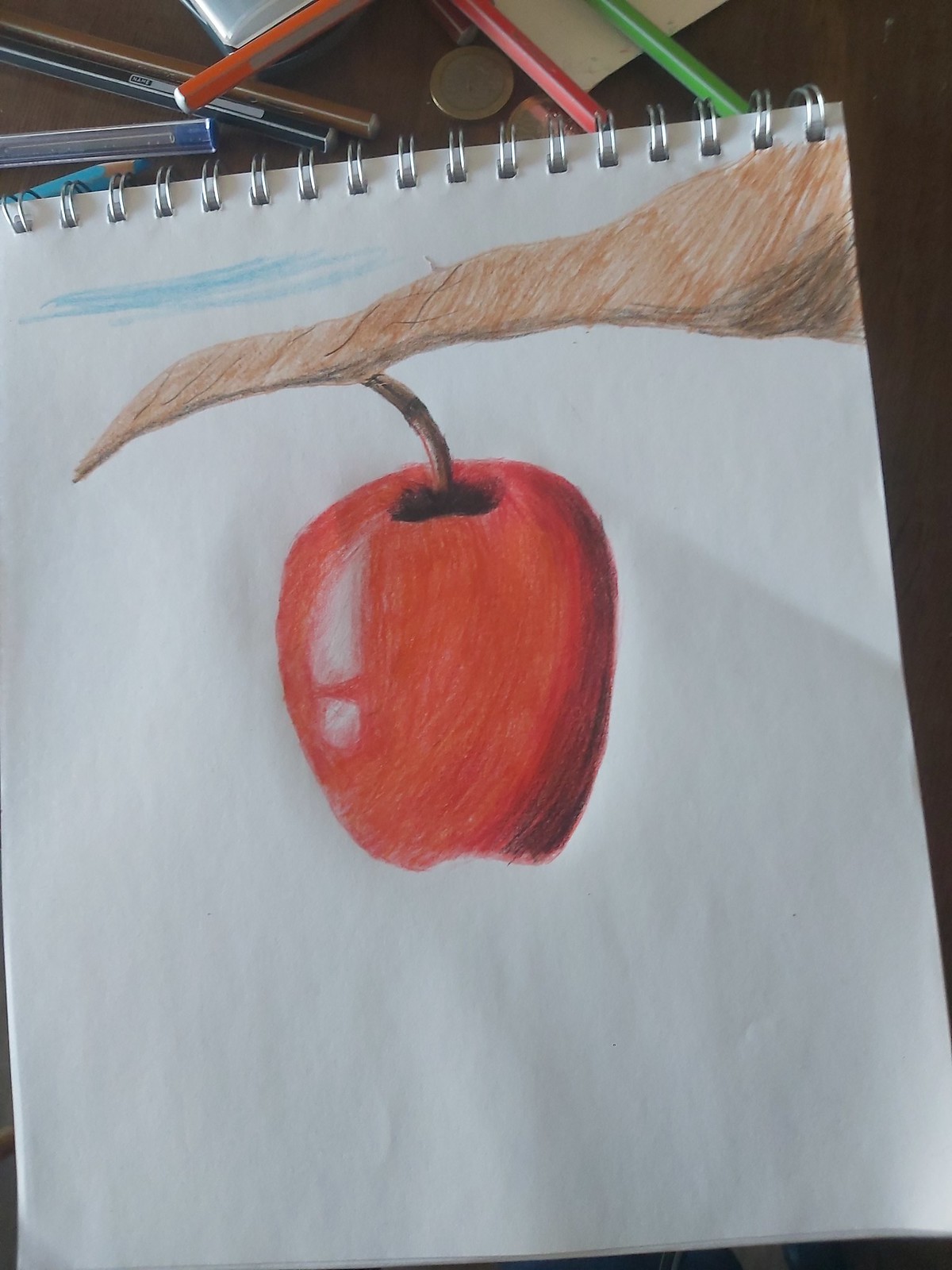This photograph features a spiral-bound notebook occupying most of the frame, lying open on a dark brown table. The notebook's white paper displays a hand-drawn illustration of a tree branch rendered in brown with a single red apple hanging from it. The artwork is created using colored pencils, giving it a slightly scratchy and untidy texture. The drawing includes detailed shading, with the underside of the branch appearing darker and the apple showcasing a shine on its left side and shadows on its right. In the top left corner of the paper, blue squiggles add an abstract element to the composition.

Scattered around the notebook are various colorful pens and art supplies in shades of blue, pink, green, orange, and more, contributing to the creative atmosphere. A shadow is cast over the piece of paper, hinting at an unseen object or light source above, adding depth and dimension to the scene.